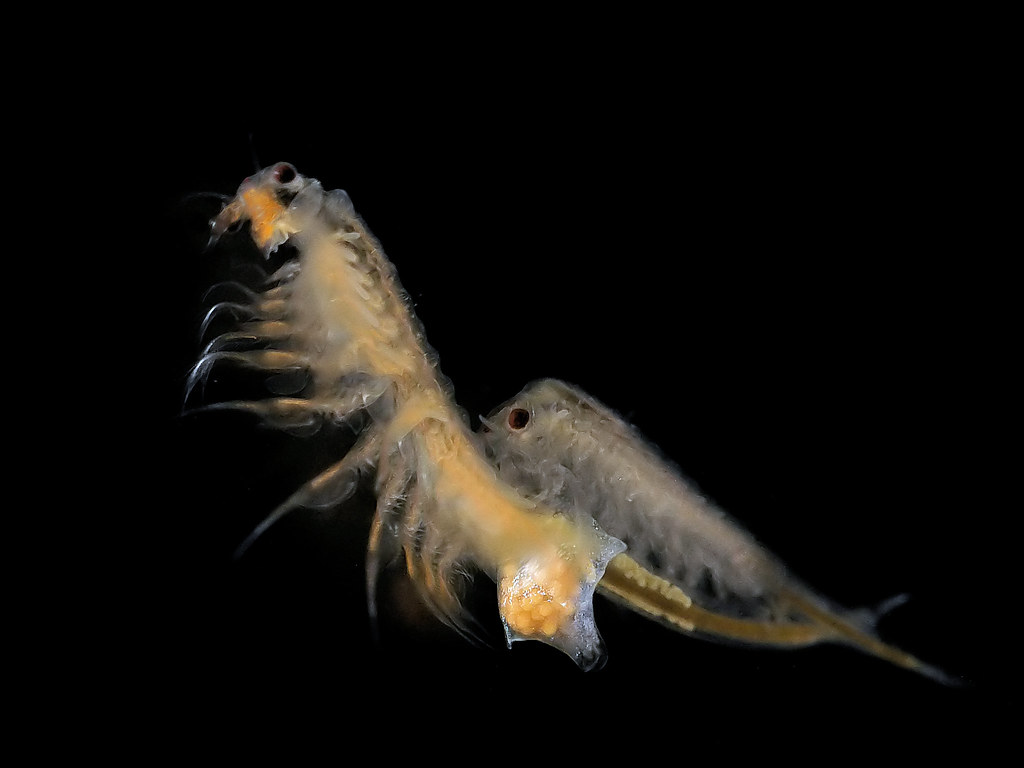The photograph showcases two translucent sea creatures floating against a pitch-black background. These creatures, which resemble brine shrimp, are positioned with the larger one on the left and the smaller one on the right. The brine shrimp on the left has a slim, slender body with an exoskeleton tinged in gray and an orange hue, multiple pointy legs, a large tail, and a beady eye. Its back has a scaly or furry texture. These creatures exhibit a unique translucency that makes them stand out starkly against the dark backdrop, highlighting their marine origins. Despite being described as reminiscent of baby lobsters or horseshoe crabs, they maintain distinct differences, especially in the body's coloration, with a more pronounced orange on the left and a clearer, more transparent appearance on the right. The image evokes a sense of augmented reality due to its strikingly detailed and almost surreal depiction of these marine organisms.